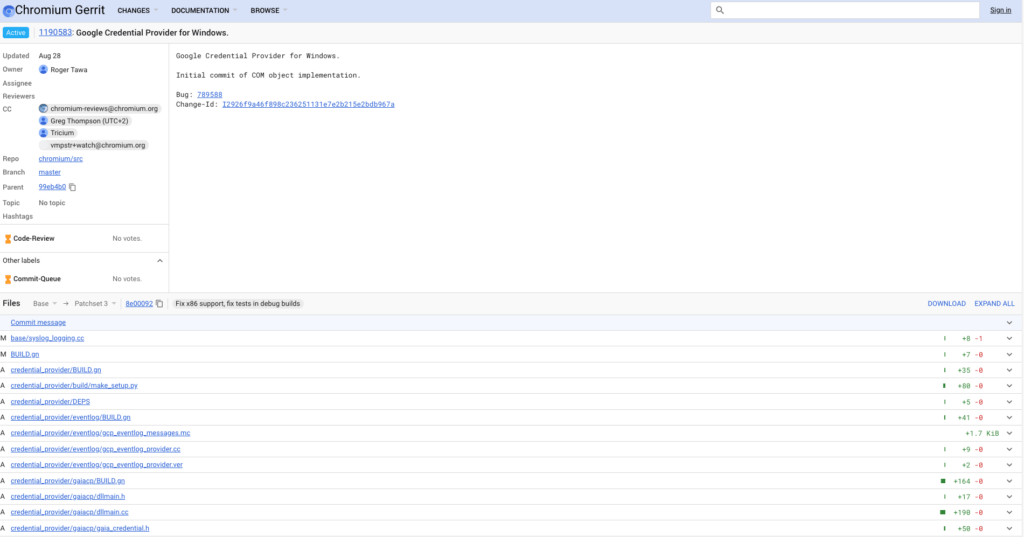The image displays a program window with various interface elements. At the very top left, the window includes tabs and labels such as "Chromium," "Garrett," "Changes," "Documentation," and "Browse," along with the numerical code "119053," and references to "Google Credential Provider for Windows." Following these, there are additional labels: "Updated," "Owner," "Assignee," "Reviews," "CC," "Repo," "Branch," "Parent," "Topic," and "Hashtags." A section titled "Velocis Code Review" appears, followed by "Common Queue" and "Files," with a list containing several blue file names, some marked as "Confidential."

To the far right side of the interface, there are options for "Download," "Expand All," and "Blue Text." The overall layout resembles that of a software or code review program window. In the top right corner, there's a white search bar featuring a magnifying glass icon on the left side and an underlined sign-in button with black text.

At the center, there is a title reading "Google Credential Provider for Windows" accompanied by a description: "Initial Commit of Com, Object, Implementation, Bug, Sub, Something, Change, HID." On the left side, it shows the update date ("Updated: August 28th"), the owner's name ("Roger Something"), and review details ("Review, CC, His Something .org"). Names such as "Greg Thompson" and "Trisium" are present, though slightly out of focus and difficult to read clearly.